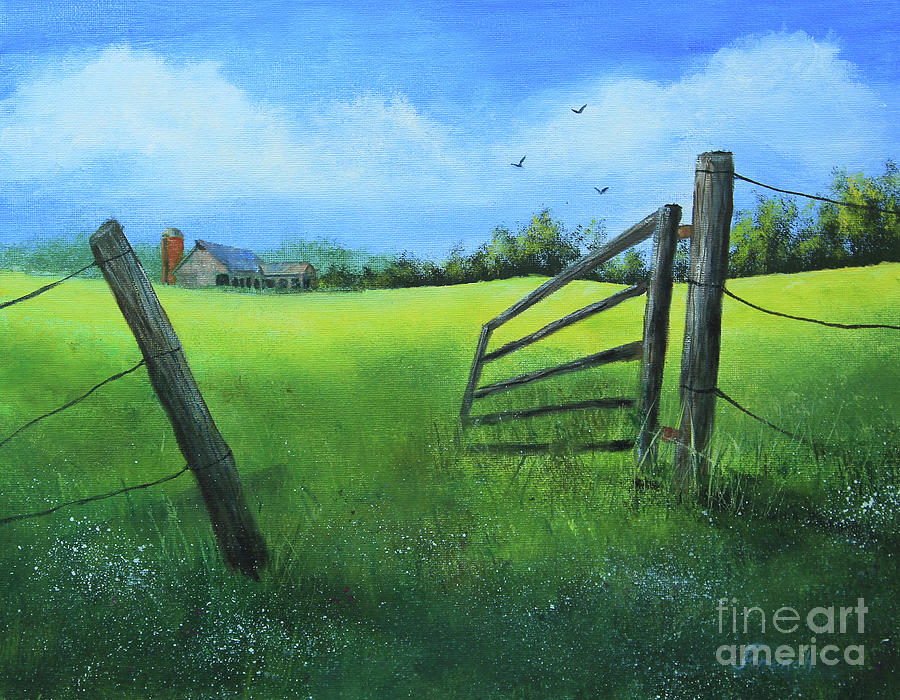This painting depicts a serene country scene centered on a dilapidated wooden fence gate, which looks as though it's about to fall off its broken hinges. The fence gate, dark gray or brown, stands diagonally connected to a dark green post on the right side, set amidst a lush green field that transitions from dark green at the bottom to a lighter, lime green toward the background. Clustered on the right side are three wires probably meant to keep animals out.

In the background, a row of dark green trees marks the boundary of the farm. Nestled among these trees stands an old farmhouse with a blue roof and several identical small doorways or windows, suggesting it might partly serve as a stable. Beside the farmhouse, directly behind it, is a red or brown wooden silo with a rounded metal top.

The sky above is a vibrant blue, dotted with big, fluffy white clouds and three birds in flight. On the left side of the field lies a suburban-looking house flanked by a small orange building. The overall impression is of a classic country setting, enhanced by the presence of scattered little white flowers in the front.

Adding a modern touch, the painting is imprinted with "Fine Art America" in the bottom right corner, likely indicating the art distributor. Despite the rundown elements like the broken fence, the scene radiates a timeless beauty and tranquility.